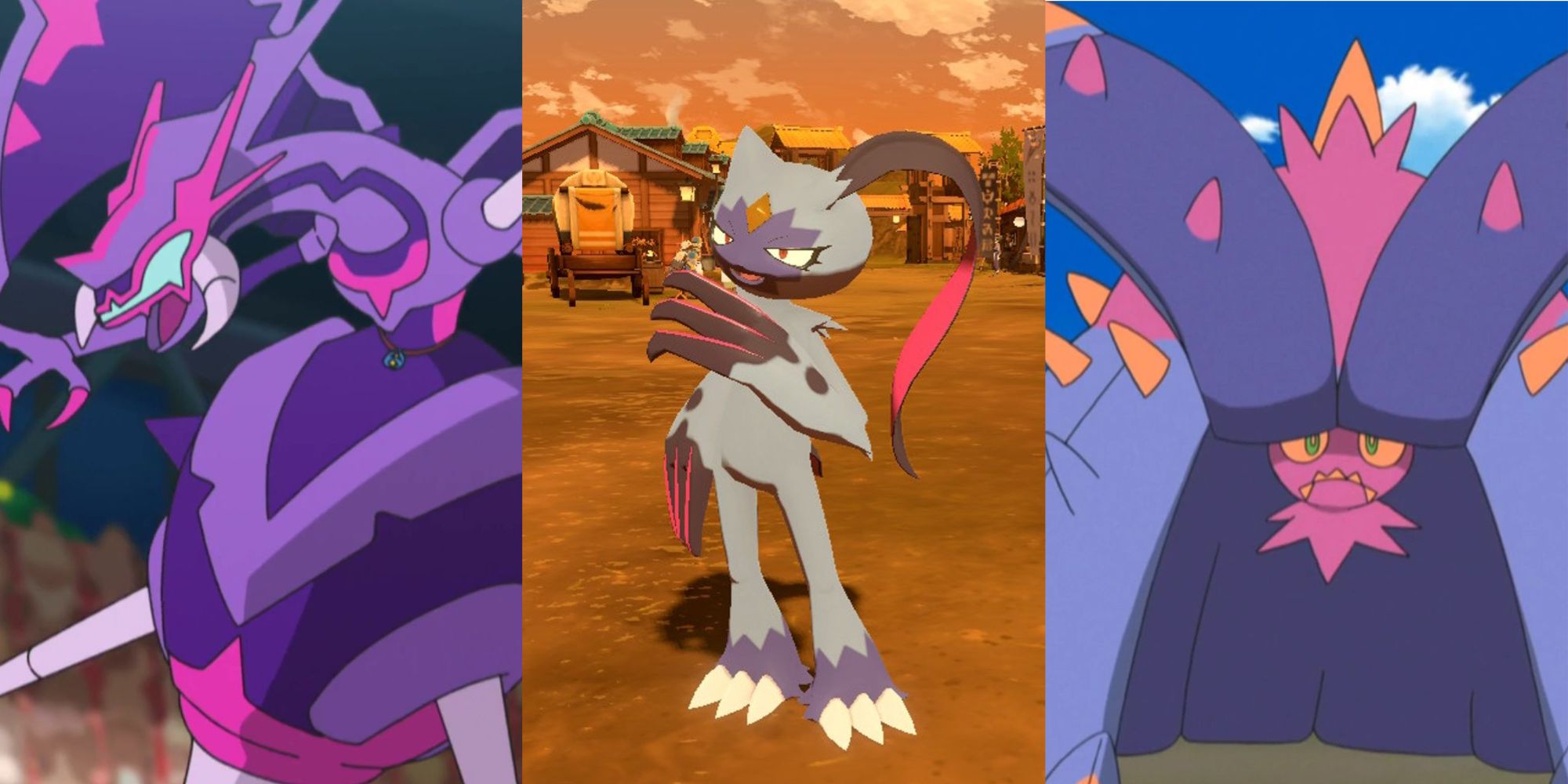The image is a triptych comic featuring three distinctive, anthropomorphic cartoon creatures. In the first panel on the left, there's a close-up depiction of a dragon-like creature with a large purple body adorned with shades of light purple, dark purple, and pink. It has a long arched neck, a small head, white fangs, and purple claws with pink nails, partially covered by an object resembling a blue visor-like helmet.

The middle panel showcases a gray cat-like character standing upright, facing the viewer. This character is in a fantasy setting with an orange and brown background, featuring orange clouds and a house or old-fashioned wagon. The cat has a purple starburst around its face, a yellow diamond on its forehead, purple around its toes, exaggerated white claws, and long brown fingernails, extending from its paw-like hands. A long ponytail transitions from brown at the top to pink and purple down its length.

In the rightmost panel, a frowning creature with a tiny pink face and green eyes seems to be trapped within a setup involving elaborate structures. It has large purple and pink horn-like tentacles emerging from its head, and the background is a blue and darker blue gradient with orange and pink triangular patterns. The creature's body is gray, and it appears to be encased in what looks like a blue and purple skirt with a green underside, accentuated by purple tubes with pink triangles.